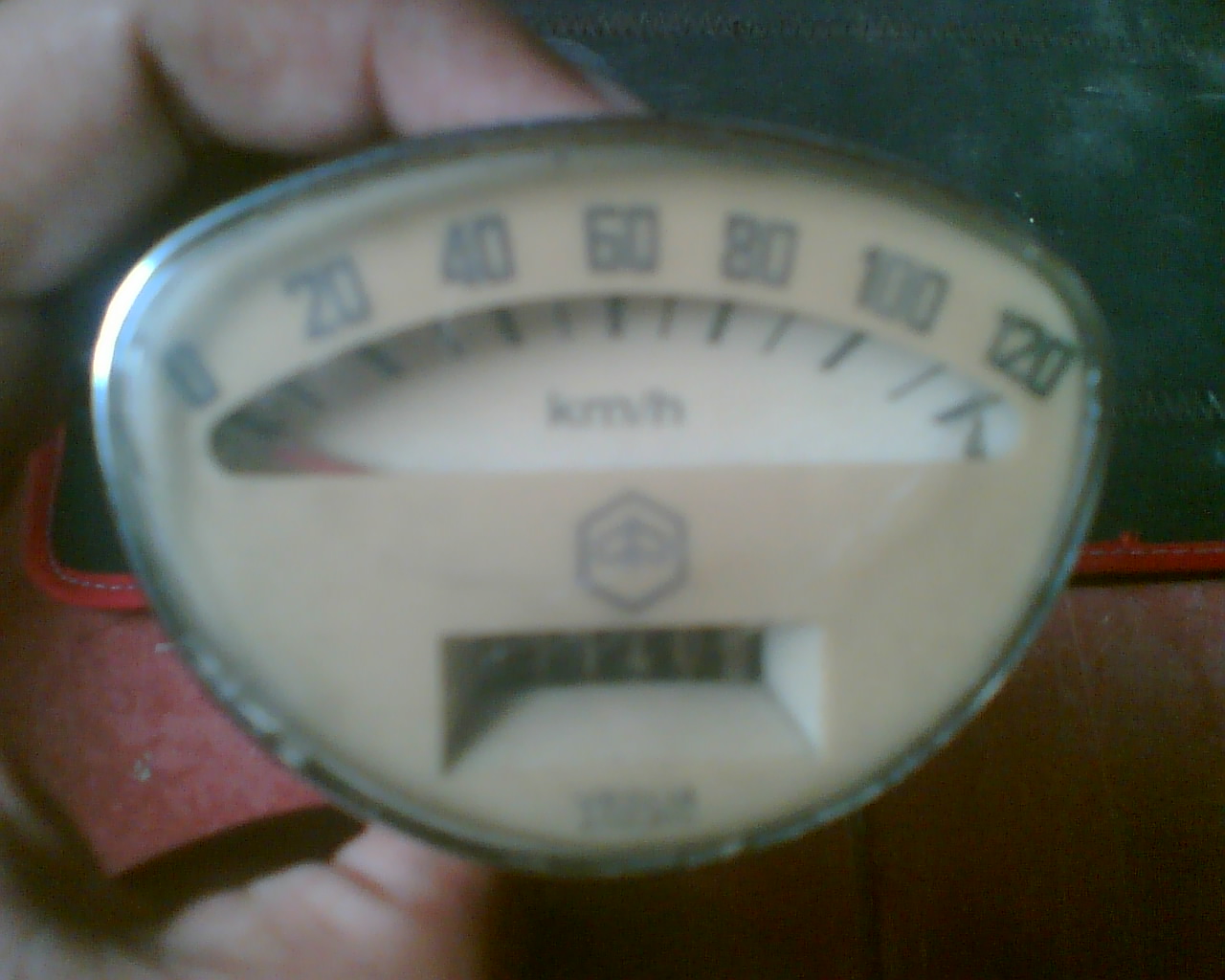This horizontal rectangular photograph, slightly blurry, captures a vintage handheld gadget centrally placed. The device, featuring a cream-colored body bordered by silver, has a rounded top and bottom with longer sides. Along its upper edge, dark-font numbers are arranged sequentially: 0, 20, 40, 60, 80, 100, and 120. Beneath these numbers, a white dial is present. The dial is marked with fine black lines radiating outwards like minute hands on a clock, creating an intricate pattern. A small red pointer line extends from the center, and there is a notation of "km/h."

Further down the cream-colored body, there’s an emblem followed by what appears to be a counter. A hand, visible with fingers from both the top and bottom, securely holds the device. The hand on the left side is adorned in red fabric, featuring a bright red edge with a darker red material inside, boasting noticeable stitching along its edge. This red fabric continues from the center bottom to the middle right side of the image. The background contrasts with a green fabric, also marked by green stitching, enhancing the overall color dynamics of the photograph.